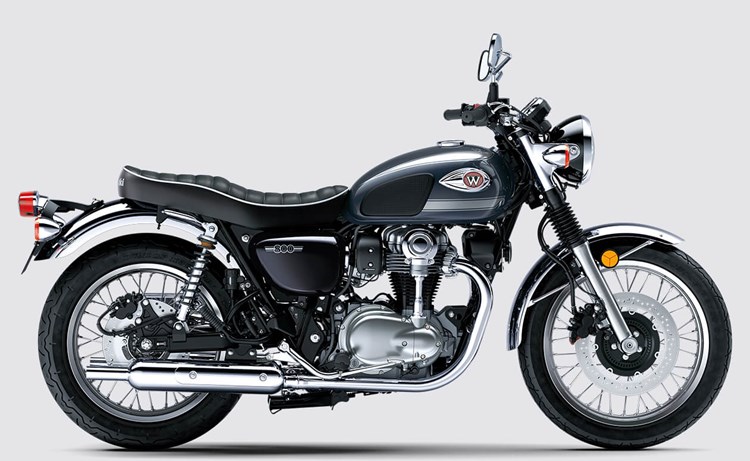This image features a sleek, brand-new black and blue motorcycle with a metallic bluish tint on the gas tank, adorned with a small "W" emblem on a red circle. The bike appears pristine, with no signs of road wear or dirt, indicating it has likely never been ridden. Its design is elegant and streamlined, boasting chrome accents on the muffler, inner parts, and fenders. 

The motorcycle is equipped with standard handlebars, complete with round rear and side view mirrors. Safety features include an orange safety reflector on the front fender and a red taillight at the back, accompanied by an additional orange taillight. The front fork features accordion-style shock protectors, adding to its polished look. 

A long double seat suggests ample room for both a rider and a passenger. The motorcycle displays a 500 designation on the engine case beneath the seat. The photo, taken against a plain white background, showcases the bike in a standing position without the assistance of a kickstand or support. Overall, it encapsulates the aesthetic of a stylish and modern ride, predominantly in black with chrome highlights, exuding a sense of sophistication and functionality.